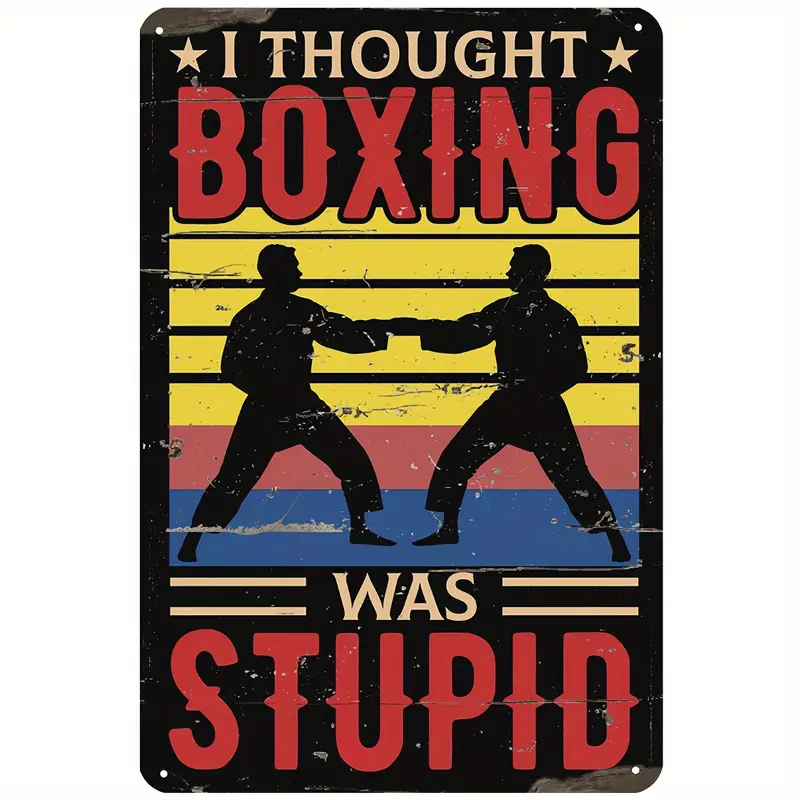This image is a stylized, weathered sign featuring a background that resembles horizontal planks in yellow, red, and blue. Centered are two black silhouettes, seemingly male, positioned in mirrored martial arts stances, likely wearing traditional karate gear. At the top of the sign, flanked by stars, is the phrase "I thought," followed by "boxing" in bold red letters with a black outline. Below the figures, the text continues with "was" set in yellow and "stupid" in large bold red letters. The sign has holes in all four corners, indicating it is meant for wall-hanging.